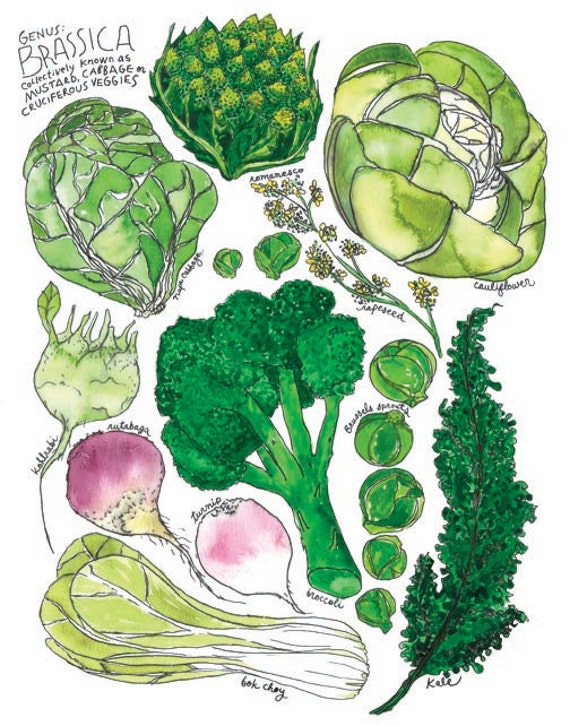This image features a white background with detailed illustrations of various cruciferous vegetables, all belonging to the genus Brassica, collectively known as mustard, cabbage, or cruciferous veggies. The text, appearing as handwritten in black, is positioned in the upper left corner and reads: "genus Brassica, collectively known as mustard, cabbage, or cruciferous veggies." 

The colorful illustrations are drawn in a cartoon style and are not hyper-realistic but still well-executed. The dominant colors are various shades of green, with accents of yellow, white, and a light purplish rose color. 

Starting clockwise from the top, the imagery includes romanesco with a spiral pattern, yellow, white, and green cauliflower, rapeseed, rich green kale, bright green broccoli, Brussels sprouts, bok choy, and purplish kohlrabi. Centered in the image are napa cabbage and green and white turnips along with rutabaga. The vegetables all showcase the diverse yet related members of the Brassica family.